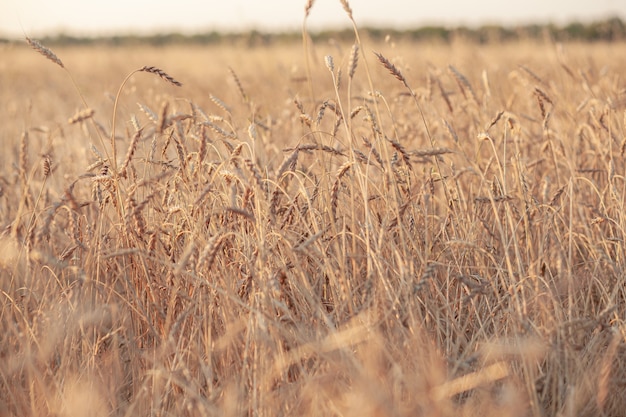The image captures an expansive field of wheat under the afternoon sun. Focused prominently in the middle, the golden grain stalks stretch upwards, with their lower parts blending into a sea of tan hues. The bottom of the image shows blurred stems, adding depth to the scene. At the top, a thin strip of sky peeks through, framing the endless field that seems to merge into a distant line of green trees. The tops of the wheat stalks are darker, contrasting against the lighter shades below. This close-up view highlights the varying shades of wheat and conveys a sense of calm and vastness, illustrating the boundless beauty of the countryside.